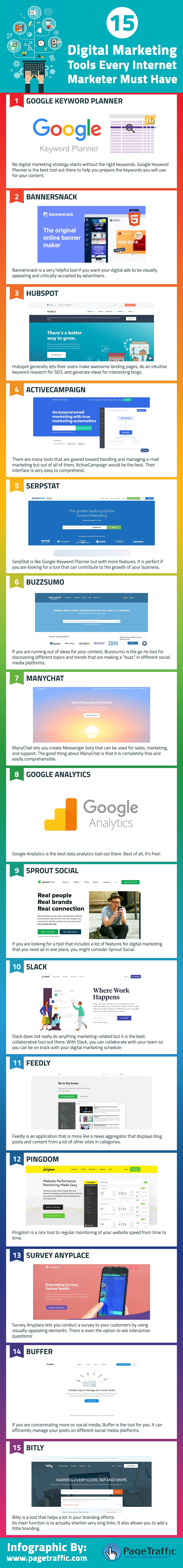The image is a screenshot, likely taken from a cell phone, given its portrait orientation and proportions which are about three times taller than it is wide. The top of the screen features a light blue horizontal border. Below this border is an image of a black and brown pillar-like object with gray bubbles emanating from it, containing indistinguishable items. Adjacent to this object is a white circle with blue font displaying the number '15'. Underneath the circle, white text reads "Digital Marketing," followed by an unreadable font, and then "Marketer Must Have."

The screenshot continues downward, bordered by a vibrant rainbow gradient that starts with red at the top and transitions to violet at the bottom on both the left and right sides of the image. Horizontally aligned white text boxes are arranged vertically down the screen, each separated by a border that follows the same red-to-violet color gradient. The first text box features the word "Google" accompanied by an image. Following this are several other images and objects that are too small to discern clearly but appear to be color-coded in alignment with the spectrum of colors present in the border.